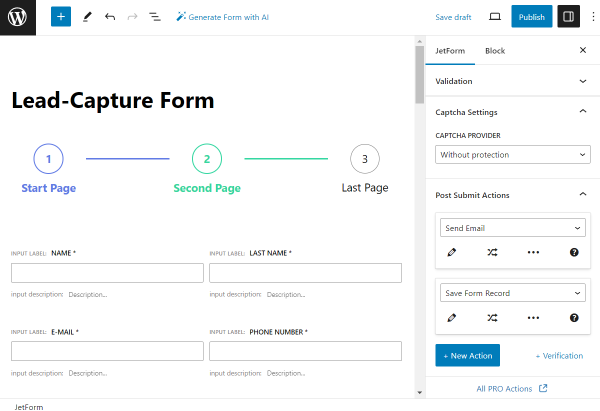The image depicts a webpage interface designed for generating forms using AI. At the top, there is a distinctive logo: a white "W" within a white circle set against a black background. Beside it, notable icons include a blue box with a plus sign, a crayon, two arrows, and diagonally oriented lines. The primary heading reads "Generate Form with AI," in blue text, directly above a subheading, "Lead Capture Form."

The form creation process is visually outlined in three stages. The first stage is indicated by "Start Page" in blue text and a blue circle containing the number "1," followed by a blue line. The second stage is labeled "Second Page" in green, with a green circle containing the number "2," followed by a green progress bar. The final stage is marked by "Last Page" with a circle containing the number "3."

Below these stages, there are several empty white fields for user input, including spaces for a first name, last name, email, and phone number. At the bottom of this section, there is an option labeled "Inform." Towards the right side of the interface, there are additional options. "Save Draft" appears as a clickable button, along with a blue "Publish" button. Adjacent to these, in a black bar, there is an option featuring a white icon with the text "Jet Form Block Validation." 

Further settings include "Capture Settings," detailing "Capture Provider" with a current setting of "Without Protection" in a white bar. Below this, "Post Submit Actions" has options like "Send Email" within a white bar. Additionally, there are options to "Save Form," "Record," and a blue bar indicating "New Action Verification." Lastly, a section labeled "All Pro Actions" is present underneath these settings.